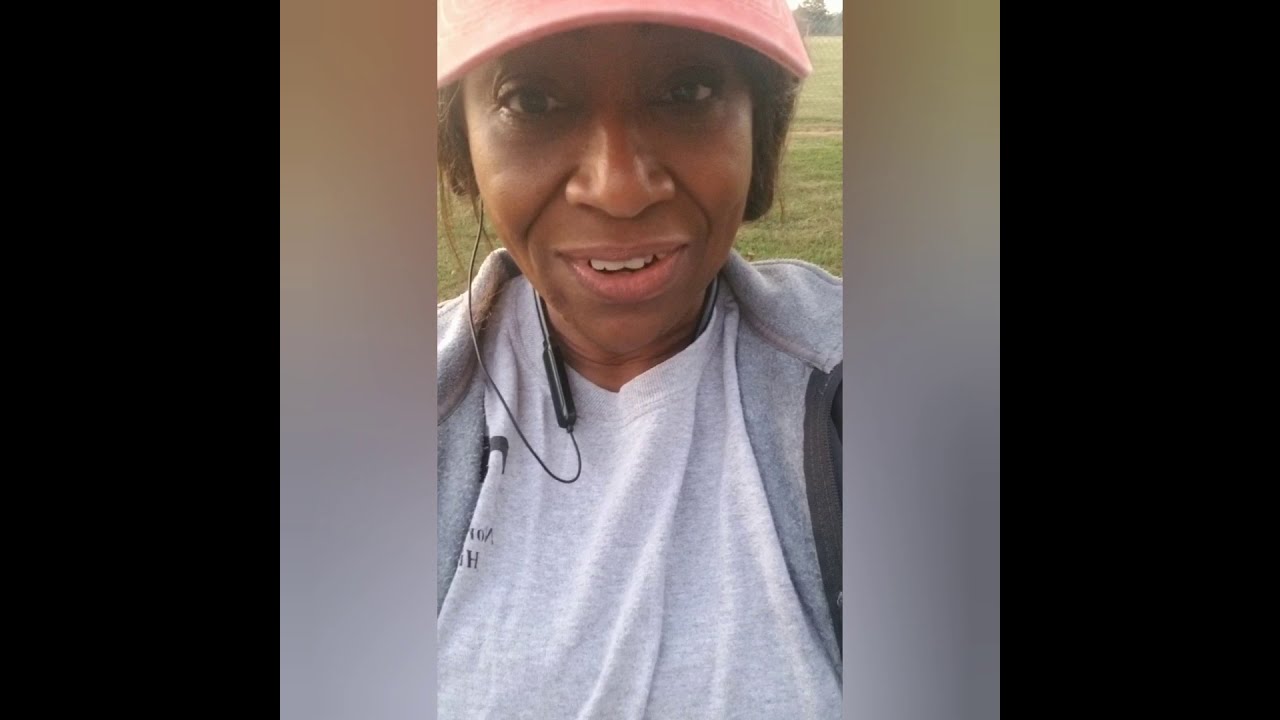The image is a horizontal rectangular selfie bordered by two thick black stripes on the left and right, and inner vertical brownish-gray stripes. It features an African-American woman looking directly into the camera with a smile, her teeth slightly exposed. She is wearing a pink baseball cap, which partially obscures her eyes, and her hair is tucked underneath it. Thin in-ear headphones with an inline volume control dangle from her ears. Her outfit includes a light grey t-shirt with some writing near the right breast pocket, covered by a dark grey hooded jacket with lighter grey accents along the zipper. Behind her, there is a mowed green field extending into the distance with trees dotting the far horizon.